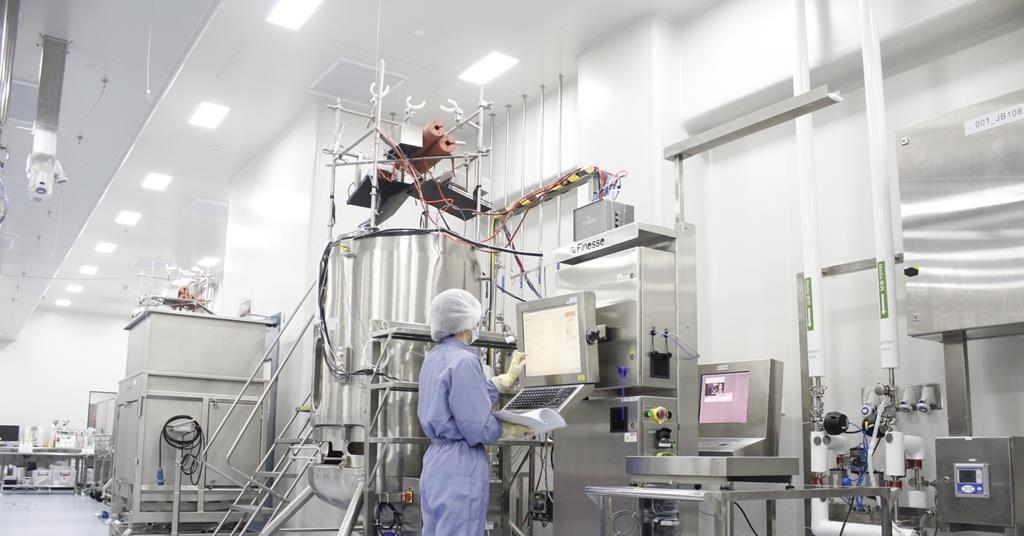This is a horizontal rectangular photograph taken inside a large, sterile lab or industrial testing facility characterized by its clean, professional environment. The dominant colors are white and silver-gray, creating a cold, clinical aesthetic, with fluorescent lights illuminating the space from the ceiling. In the center of the image, a person is standing and working at a keyboard, partially turned away from the camera. This individual is dressed in a blue jumpsuit and full protective gear, including gloves, a head covering, and a face mask, indicating a high standard of cleanliness and safety, typical of a cleanroom setting. Surrounding the person is an array of gray and stainless steel equipment, including a tall piece of machinery adjacent to them, silver vats, and additional apparatuses extending towards the back of the room. To the person's right is a computer screen setup, contributing to the impression of a complex, technologically advanced facility.